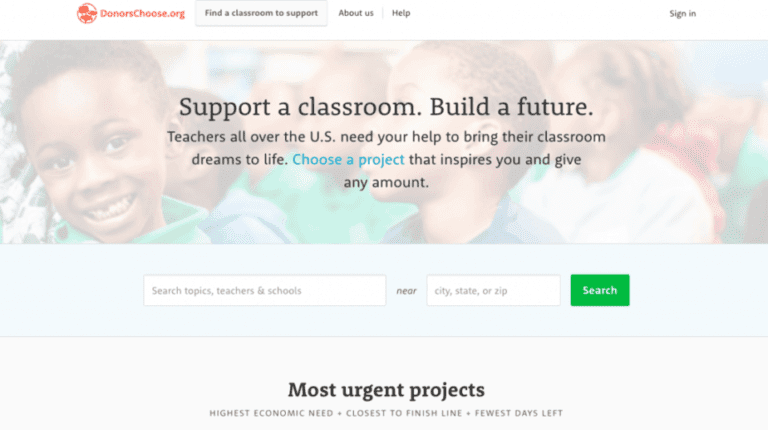The homepage of DonorsChoose.org prominently features its logo on the left. Adjacent to the logo is a button labeled "Find a Classroom to Support," indicating the current active tab. Next to it are additional tabs labeled "About Us" and "Help," with a "Sign In" button located on the far right.

The top banner displays a heartwarming photograph of young children, approximately five to six years old, smiling in a classroom setting. All eight children appear to be African American. Overlaying this image is black text that reads: "Support a classroom, build a future. Teachers all over the U.S. need your help to bring their classroom dreams to life." Directly below, a link encourages visitors to "Choose a project that inspires you to give any amount."

Underneath this call to action, a search bar allows users to find projects by topics, teachers, and schools, with an additional proximity filter labeled "Near." This search functionality includes fields for city, state, or zip code, and is accompanied by a green "Search" button.

Further down, the page highlights sections labeled "Most Urgent Projects" and categorizes them by "Highest Economic Need," "Closest to Finish Line," and "Fewest Days Left." This summary captures the essence and navigational structure of DonorsChoose.org's homepage.